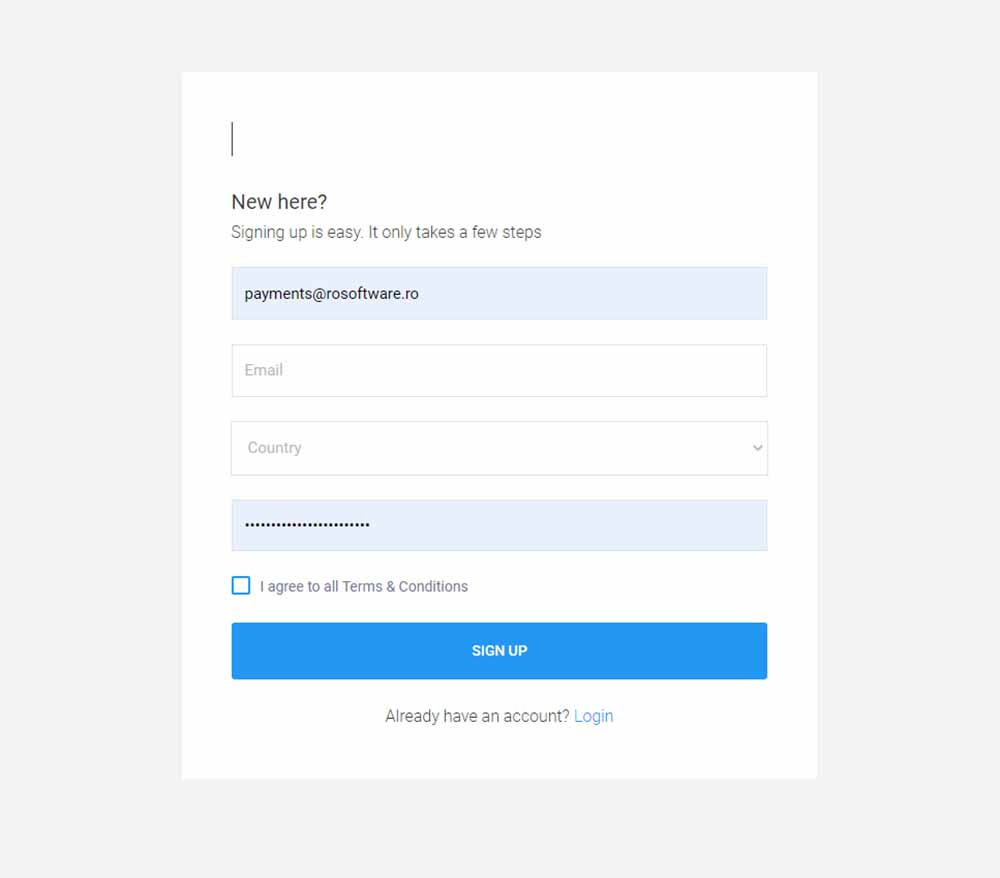The image depicts a screenshot of a website's user registration form. At the top of the form, there is a header with some introductory text, though the exact wording is unclear. Directly below this header is a thin line, possibly indicating where users can enter information.

The form starts with a prompt that reads, "New here? Signing up is easy. It only takes a few steps." An example email address, "payments@rawsoftware.ru," is already filled in at the top, suggesting either placeholder text or pre-filled content. Below this, there is a dedicated field for users to input their own email address.

Next, the form includes a country selection field with a drop-down arrow, allowing users to choose their country from a list. Further down, there is a password field where a lengthy password, approximately 15 characters long, has been entered.

Beneath the password field, there is an unchecked checkbox labeled "I agree to all terms and conditions." Finally, at the bottom of the form, there is a prominent "Sign Up" button featuring a blue background with white text.

Additionally, there is a prompt for existing users that reads, "Already have an account? Login," accompanied by a login button in blue text.

Overall, the form appears to be straightforward, guiding new users through the sign-up process while also providing an option for existing users to log in.